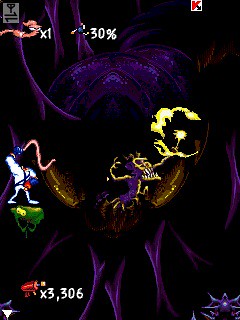The image appears to be a vibrant and surrealistic graphic, potentially from a video game, set against a stark black background. Dominating the scene is a massive purple shape, resembling either a planet or the open maw of a giant creature, which draws immediate attention. Surrounding this enigmatic purple form are various distinctive figures, each brightly colored and sharply contrasting with the dark backdrop.

On the right side, there is an unusually large-mouthed character dressed in purple, seemingly interacting with a crescent moon, which contains a small light within it, positioned near what appears to be his arm. To the left of this figure stands another character, donned in an all-white suit with a striking blue and red mask. Below this figure, a small green creature with prominent eyes, resembling a gooey slime, is noticeable.

In the bottom right corner, a symbol reminiscent of a spider adds an element of intrigue, while to the bottom left, there is a noticeable inscription of the letter "X" alongside the number "3,306." Above the central scene, a pinkish entity of unknown nature hovers, lacking any discernible facial features, adding to the image's mysterious atmosphere. At the very top, a small white square with a hint of red and a tiny arrow inside can be seen, perhaps indicating a point of focus or an interface element.